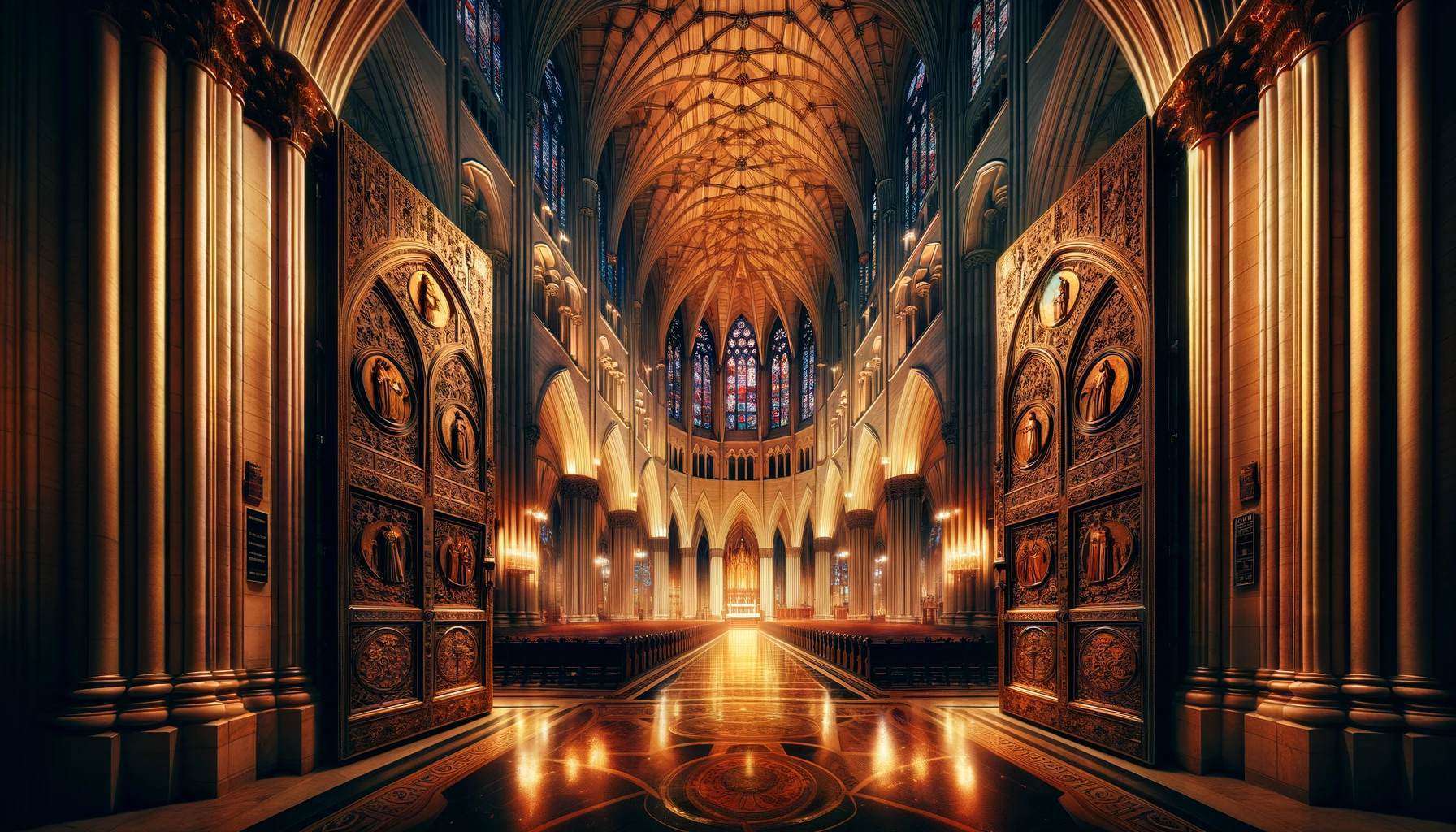This image is a highly detailed portrayal of an elaborate cathedral, possibly AI-generated or a 3D rendering. In the foreground, you see two tall and heavy carved wooden doors, swung inward, each adorned with seven oval portraits of saints or important figures. These doors lead into a grand, gleaming corridor with a highly polished floor that almost looks metallic, featuring an indiscernible design. The space is illuminated with a warm, golden hue from numerous light sources that seem to diffuse in a hazy, almost unnatural manner. On both sides of the corridor, small, tightly spaced wooden pillars add to the intricate interior, leading back through rows of pews towards a distant, bright golden altar. The walls and ceiling are adorned with stained glass windows, which cast vibrant red, white, and blue hues throughout the space. The ceilings feature a complex arrangement of arched stone pillars and archways, contributing to the cathedral's majestic and somewhat surreal appearance.